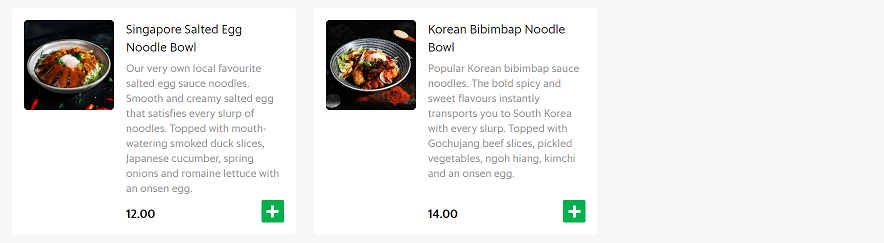This image is a screenshot from a restaurant's website showcasing some of their menu items with detailed descriptions and accompanying photos. Each item is presented within a white square, featuring a small picture in the top left-hand corner.

In the first square, the dish is identified as the "Singapore Salted Egg Noodle Bowl." The accompanying photograph displays a metal bowl filled with a variety of ingredients, predominantly green in color. The description reads: "Our very own local favorite, salted egg sauce noodles. Smooth and creamy salted egg sauce that satisfies with every slurp. Topped with mouth-watering smoked duck slices, Japanese cucumbers, spring onions, and romaine lettuce, finished with an onsen egg." The price for this dish is listed as $12. Additionally, there is a small green box in the bottom right-hand corner featuring a plus sign, likely for adding the item to your cart.

The second square highlights the "Korean Bibimbap Noodle Bowl." The image also shows a metal bowl filled with vibrant ingredients. The description states: "Popular Korean sauce noodles with bold, spicy, and sweet flavors that instantly transport you to South Korea. Topped with gochujang beef slices, pickled vegetables, ngo hee yang kimchi, and an onsen egg." This dish is priced at $14 and similarly features a green box with a plus sign in the bottom right-hand corner for easy addition to your cart.